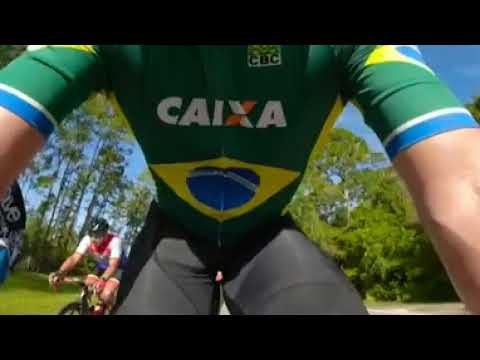Title: *Brazilian Cyclist*

The photograph captures a dynamic scene centered on a male cyclist wearing black stretch pants and a distinctive green cycling jersey adorned with blue and yellow trims, and white stripes. Emblazoned across his chest is the word "Caixa" along with a blue globe, inspired by the Brazilian flag, featuring a green stripe and a yellow diamond background. This cyclist is leaning forward with his arms on either side of the handlebars, suggesting active motion, possibly within a race. Mounted on his handlebars is what appears to be a camera, capturing the thrilling experience.

In the background, the scene reveals lush greenery and a pristine blue sky, indicating it's a sunny day. To the left of the main cyclist, another rider is visible, wearing a black helmet, a white and red top, and orange shorts. This second cyclist appears in a more full-body view and is slightly ahead, perhaps leading the race. Both cyclists seem to be in excellent physical condition, navigating through a forested area filled with green foliage.

Overall, the image exudes energy and the spirit of competition, with vibrant natural colors of blue, green, and hints of other hues blending seamlessly into the outdoor setting.